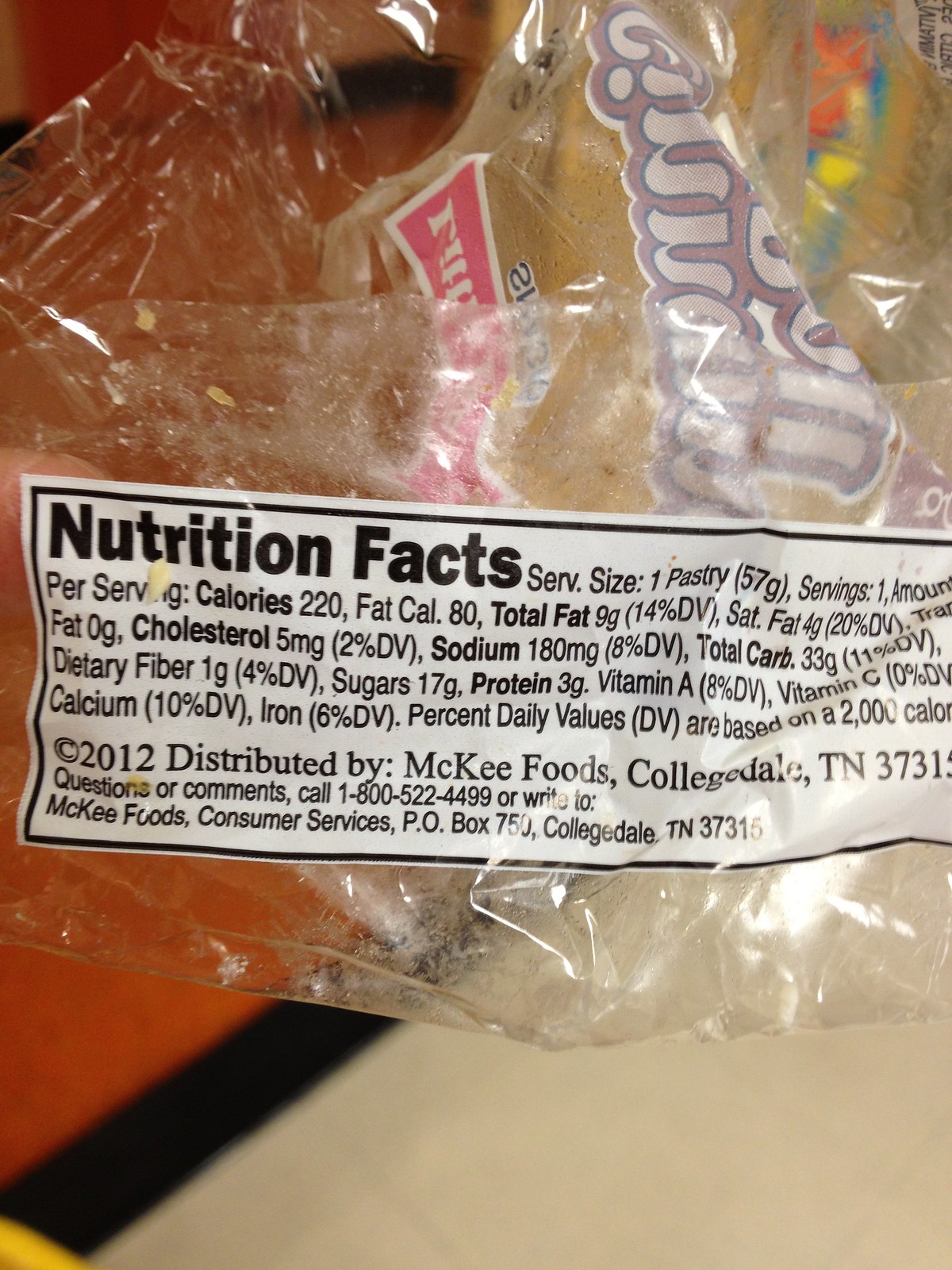This image is a detailed, close-up photograph of a clear, crinkly plastic wrapper that once contained a snack, likely a Little Debbie cinnamon roll. The plastic is transparent with some labeling visible through its folds, including a partial view of the red "Little" emblem often associated with Little Debbie products. The wrapper features a prominently displayed Nutrition Facts label with a white background and black text, bordered by a black outline. The serving size is listed as one pastry (57 grams), with a total of 220 calories per serving. The detailed nutritional information includes 80 calories from fat, 9 grams of total fat (14% DV), 4 grams of saturated fat (20% DV), 5 milligrams of cholesterol (2% DV), 180 milligrams of sodium (8% DV), 33 grams of total carbohydrates (11% DV), 1 gram of dietary fiber (4% DV), 17 grams of sugars, 3 grams of protein, 8% DV of Vitamin A, 0% DV of Vitamin C, 10% DV of calcium, and 6% DV of iron. The product was distributed by McKee Foods, with copyright information dating to 2012, based in Collegedale, Tennessee. Contact details are provided for consumer services. The packaging is shown lying on a surface, possibly a tile floor, indicated by visible lines and an orange tint in front of it. The background behind the Nutrition Facts label is white, with additional black and white text providing further product and distribution information.